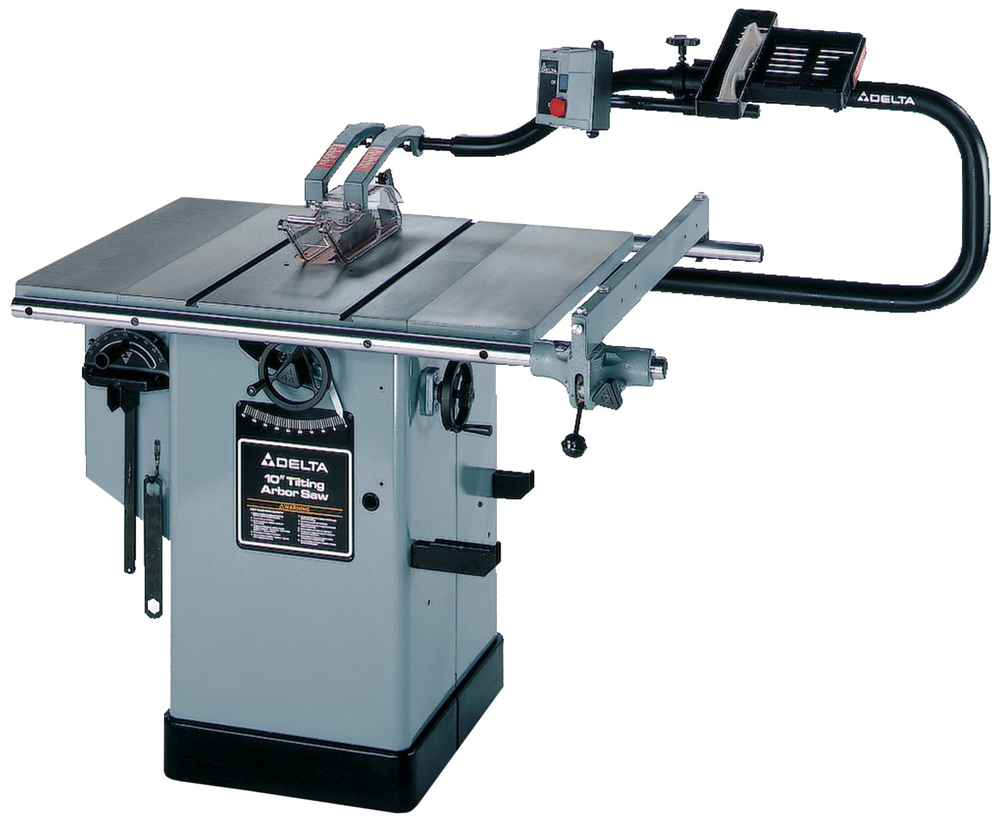The image depicts a large piece of industrial electrical equipment, specifically a Delta 10-inch tilting arbor saw. The machinery is primarily a bluish-gray color with some black components. The main structure consists of a rectangular base that supports a table-like surface. Off to the side, there is a protruding arm that loops back and connects to the table. This arm and the base feature the Delta brand emblem, which is composed of three triangles forming a larger triangle, along with the label "10-inch tilting arbor saw."

The equipment is intricately designed, with various adjustment wheels and levers on both the right and left sides for modifying the position and size of the saw blade that emerges from the top of the table. The black arm extending over the saw blade appears to have buttons, the purpose of which is not entirely clear. The overall structure includes a substantial stand that holds the machinery, with portions of it being surrounded by metal. The stand itself is gray with a black base and additional structural elements on the left side.